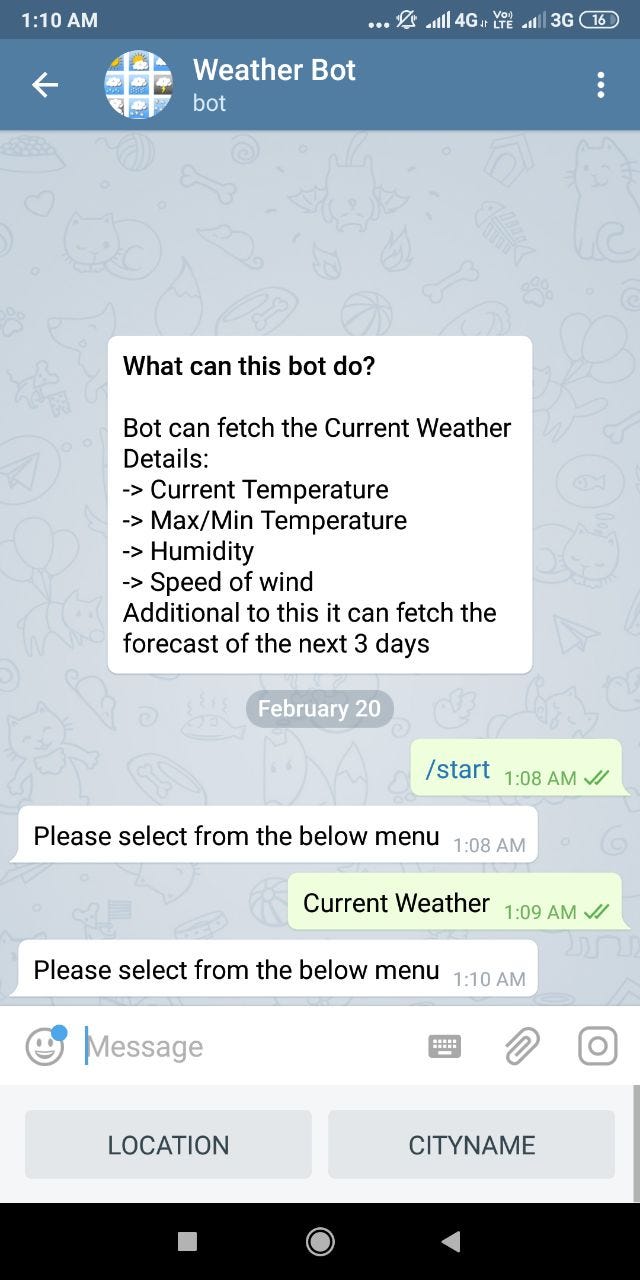This is a detailed screenshot of a smartphone displaying various UI elements at 1:10 AM. At the top of the screen on a dark blue background, the status bar contains the time on the left. To the right, there is a blue space followed by three vertical dots, indicating more options, and a notification bell showing no new notifications. Further to the right, there are five signal bars displaying "4G" connectivity and nearby, a symbol indicating "LTE". Adjacent to this, another set of three signal bars is visible, marked with "3G", and there is a "16" inside a bubble-shaped icon.

Below the status bar, on the left, there is a back arrow and next to it, a circular profile picture for "Weather Bot." Following this, the text "Weather" is displayed above the word "Bot". On the right side of "Bot", there are three vertical dots for additional options. 

The middle section features a white square on a light blue background, which reads: "What can this bot do? Bot can fetch the current weather details, current temperature, max/min temperature, humidity, speed of wind. Additionally, it can fetch the forecast of the next three days." 

Below this informational section, there is a gray button labeled "February 20" in white letters. To the right and below "February 20", a light green bubble containing "Start" in blue text is visible, next to a timestamp reading "1:08 AM". 

Further down, a white bubble with black text instructs, "Please select from the below menu", and right below it, another light green bubble reads "Current Weather". Subsequently, another white bubble repeats, "Please select from the below menu."

At the bottom of the screen, a field labeled "Location and city name" is displayed, accompanied by the standard navigation buttons of the phone.